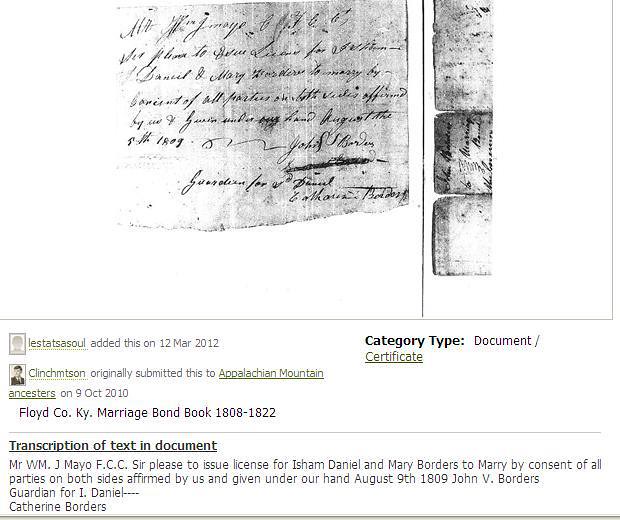The image is a screen grab from a website, showing a black and white photocopy of a worn, old-fashioned document with handwritten pen script. The document is a piece of paper, likely a marriage bond certificate dated August 9, 1809. The writing requests Mr. W.M.J. Mayo, FCC, to issue a marriage license for Isham Daniel and Mary Borders, noting it is by consent of all parties and signed by John V. Borders, guardian for I. Daniel and Katherine Borders. This photocopy is placed centrally on the webpage, accompanied by various texts explaining the document's details. Below the image, green and gray fonts detail that it was uploaded by a user named LESTA TSA SOL on March 12, 2012, and sits within the Floyd County, Kentucky marriage bond book collection from 1808 to 1822. The entire image is rectangular and slightly wide, with the main document prominently featured alongside smaller bits of additional text.